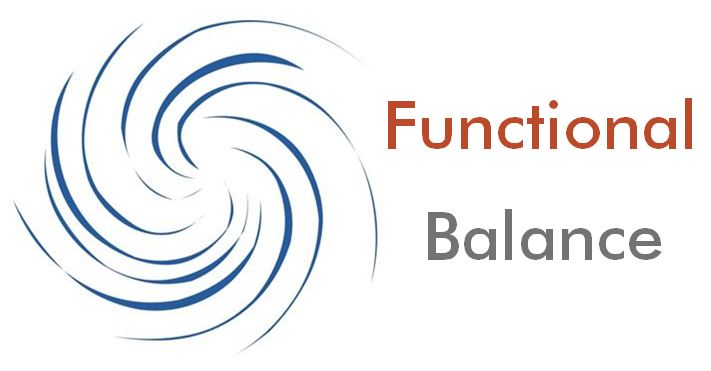The image features a logo set against an all-white background. On the left side, there is an abstract graphic resembling a swirling cyclone or fan made up of thin blue lines of varying thickness, spiraling out from a center point. This blue swirl fills the left-hand side from top to bottom. On the right side, perfectly centered, the text reads "Functional Balance" in two lines. The word "Functional" is in a dark burnt orange color with an uppercase 'F' followed by lowercase letters. Directly below it, the word "Balance" is in a medium gray tone, starting with an uppercase 'B' and followed by lowercase letters. The entire design, both the swirl and the text, is symmetrically balanced against the pristine white background, creating a clean, minimalistic aesthetic.